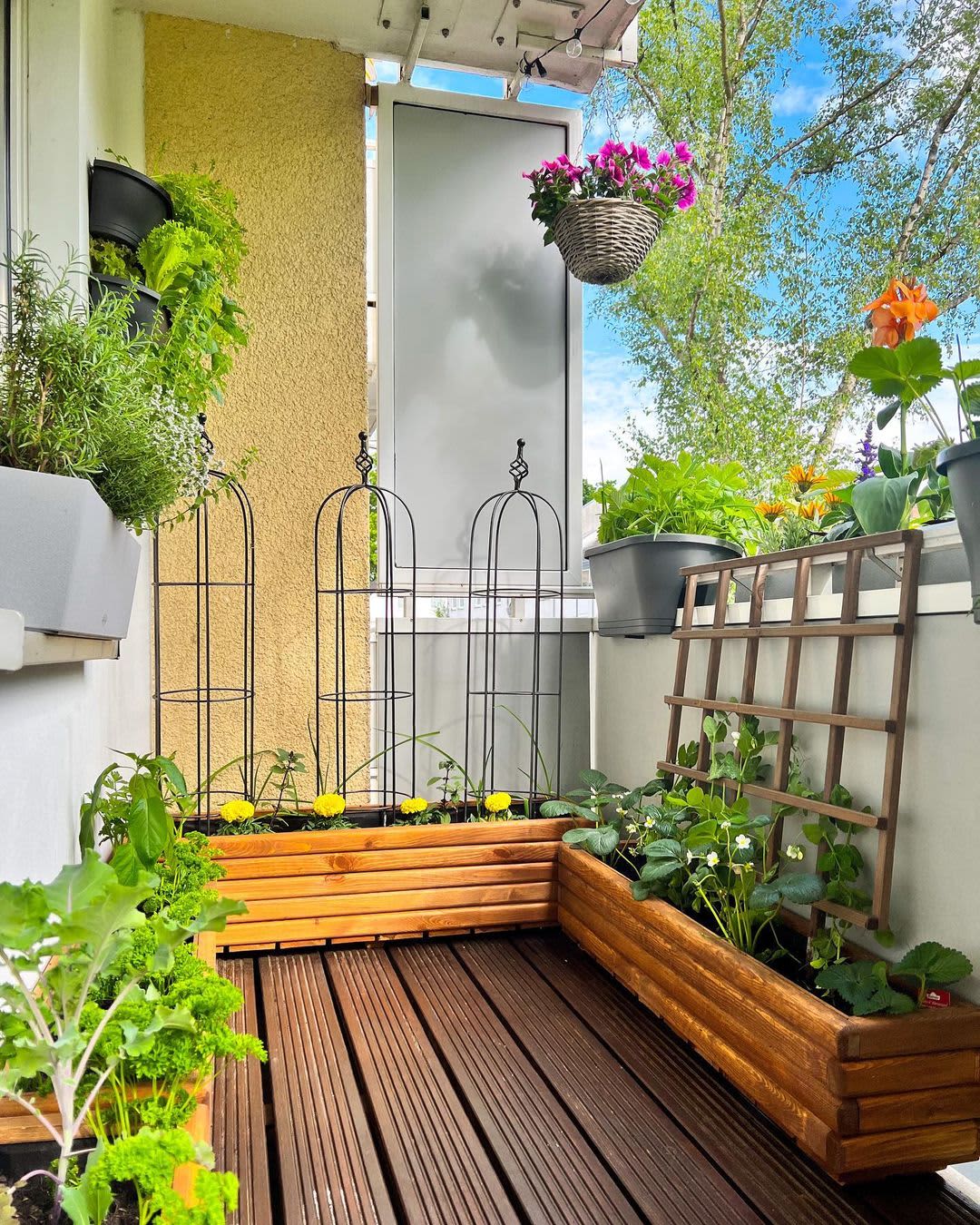The image shows a small balcony, likely from an apartment, featuring a dark wooden deck with slats through which the floor is visible. The perimeter is lined with raised flower boxes containing a variety of plants, including leafy vegetables and colorful flowers like yellow marigolds. A notable feature is the multiple trellises and cages within the boxes designed to support climbing plants. On the left, a windowsill holds additional plant containers brimming with greenery. A hanging basket filled with vibrant purple flowers is prominently displayed, and another flower basket overflows with green foliage. Beyond the plant-laden balcony, the scene opens up to reveal a blue sky dotted with white clouds and the tops of tall, green trees swaying gently under the shining sun. It is clear that the balcony owner is deeply engaged in gardening, bringing a lush, verdant touch to their outdoor space.